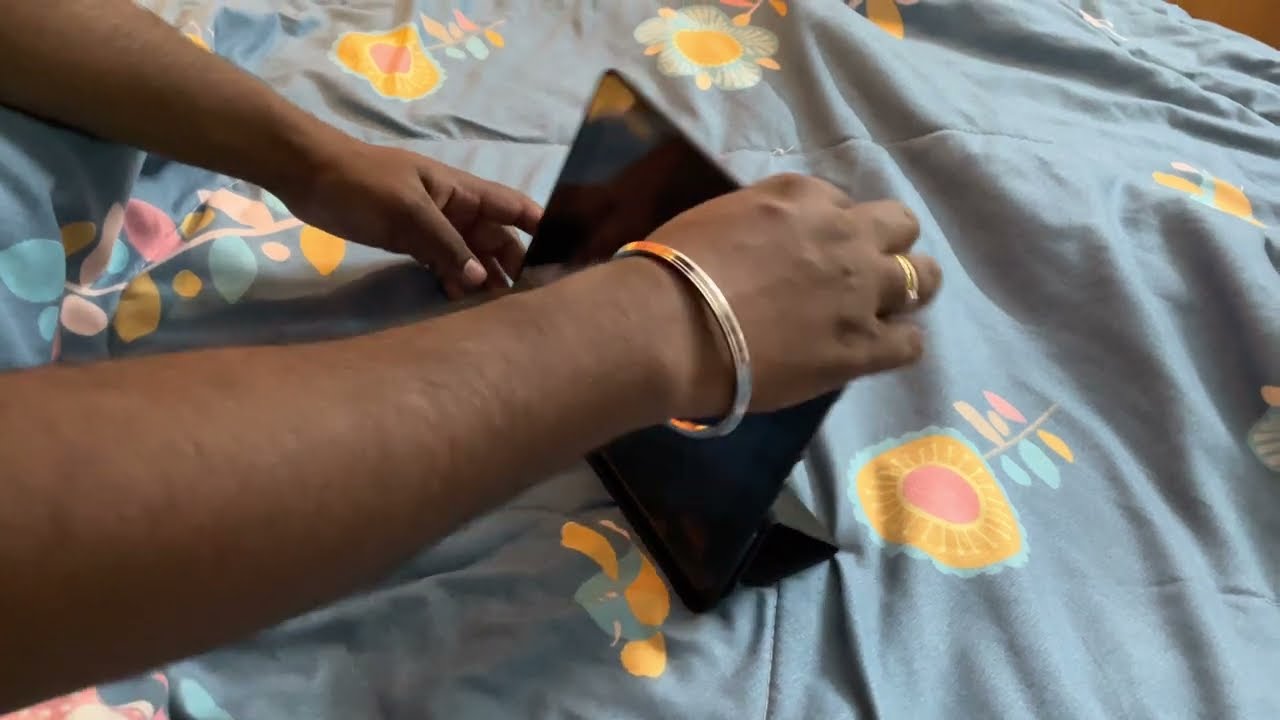This indoor photograph captures a close-up view of a black tablet being propped up in its holder atop a light blue bedspread adorned with a colorful, intricate floral pattern. The bedspread features orange, pink, and blue flowers with yellow and pink accents, along with blue and gold birds in mid-flight. Emerging from the lower left and upper left corners of the image are two forearms and hands, seemingly female, with brown skin and pink-painted nails. Gold rings adorn the right-hand ring finger, and a gold bangle circles the right wrist. The person is using both hands to steady the tablet, which reflects part of the bedspread. The device is positioned against its stand, though it appears to be off, or the screen is not clearly visible.